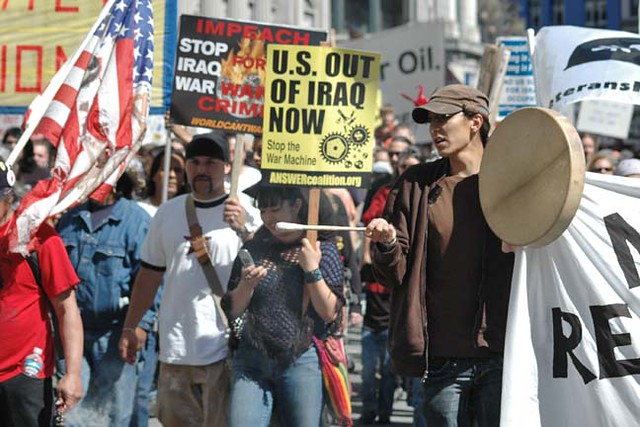The photograph captures a peaceful protest unfolding on a street with a diverse crowd holding up a variety of signs and banners. Central to the image is a woman with black hair and bangs, engrossed in her flip phone while carrying a picket sign. Her sign reads "U.S. out of Iraq now" in black text on a yellow background, followed by "Stop War Machines" and the URL "answercoalition.org." To her left stands a man in a black beanie and a white t-shirt with black edges, sporting a long black mustache and goatee. He holds a sign that says "Impeach" in red letters and "Stop Iraq for War Crimes" in white text on a black background. Next to him, partially cropped out, is an individual bearing a tattered American flag, showing signs of wear and potential burn marks. Further right in the photo, a man in a brown hat, brown jacket, and T-shirt is seen holding a makeshift drum and a stick to beat it. The crowd features people of all ages, sexes, and races, emphasizing the diversity and solidarity of the protestors. Additional signs in the background mirror the anti-war sentiment but are partly obscured by the people and other signs in the forefront. The overall scene is set outdoors, capturing the earnest and collaborative spirit of the demonstrators as they march together.